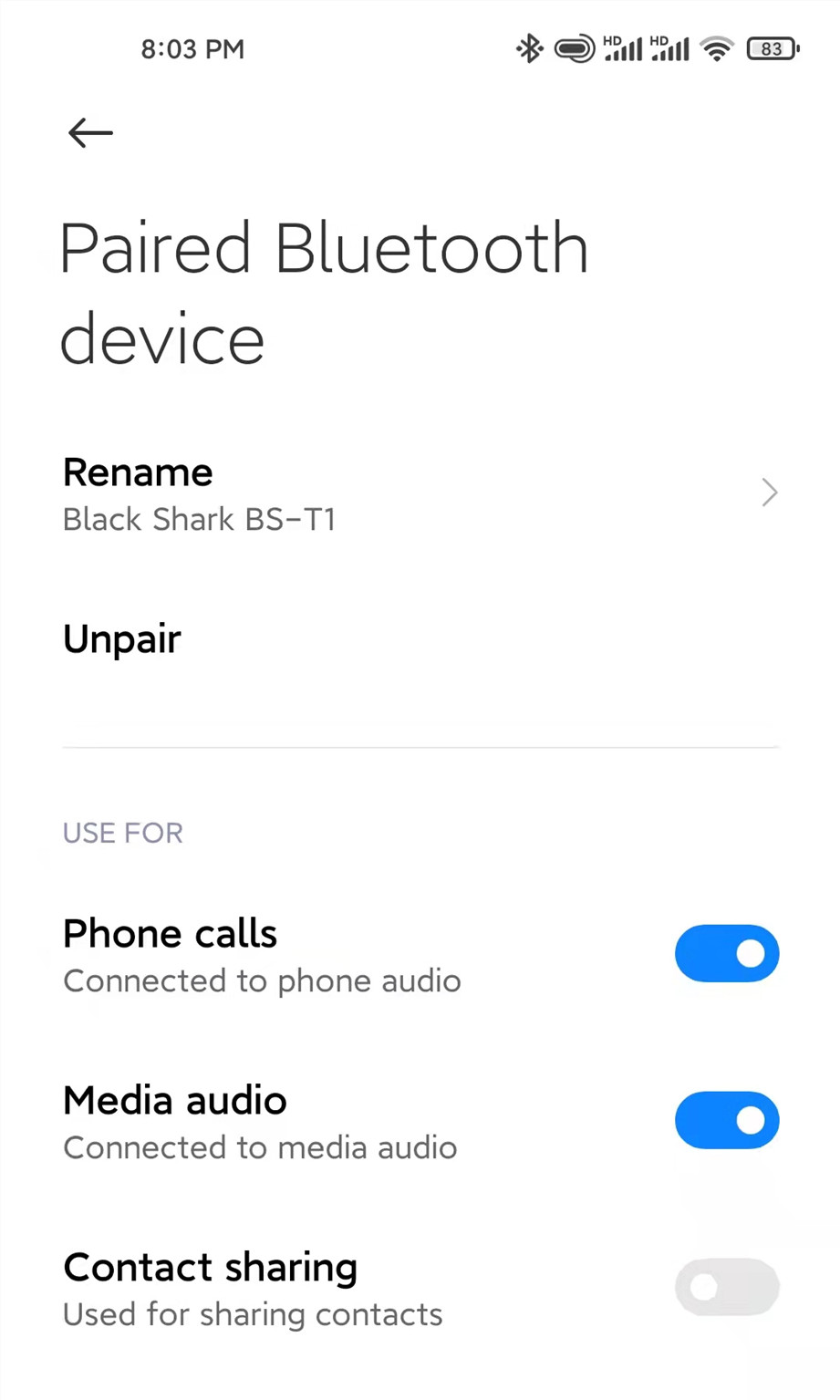The image displays a paired Bluetooth device interface. At the top, the phrase "Paired Bluetooth device" is prominently shown. Below this, there's some space, followed by the word "Rename" in bold black text. Underneath "Rename," in gray text, it says "Black Shark BS-T1."

After another section of space, the next line reads "Unpair," also in bold black text. A few spaces below that, a faint gray horizontal line spans across, dividing the page. Further down, there is a header in gray, all uppercase letters saying "Use For."

Skipping a line or two, the section begins with "Phone calls" in bold, indicating it is connected to phone audio. To its right, there's a blue toggle switch that can be used to turn this feature on or off, with a circular switch inside the oval.

Below this line, the next category is "Media audio," which is similarly indicated to be connected to media audio. Beside this, on the right, another blue toggle switch is present for enabling or disabling the feature.

After some spaces, the final section reads "Contact Sharing," which states that it is used for sharing contacts.